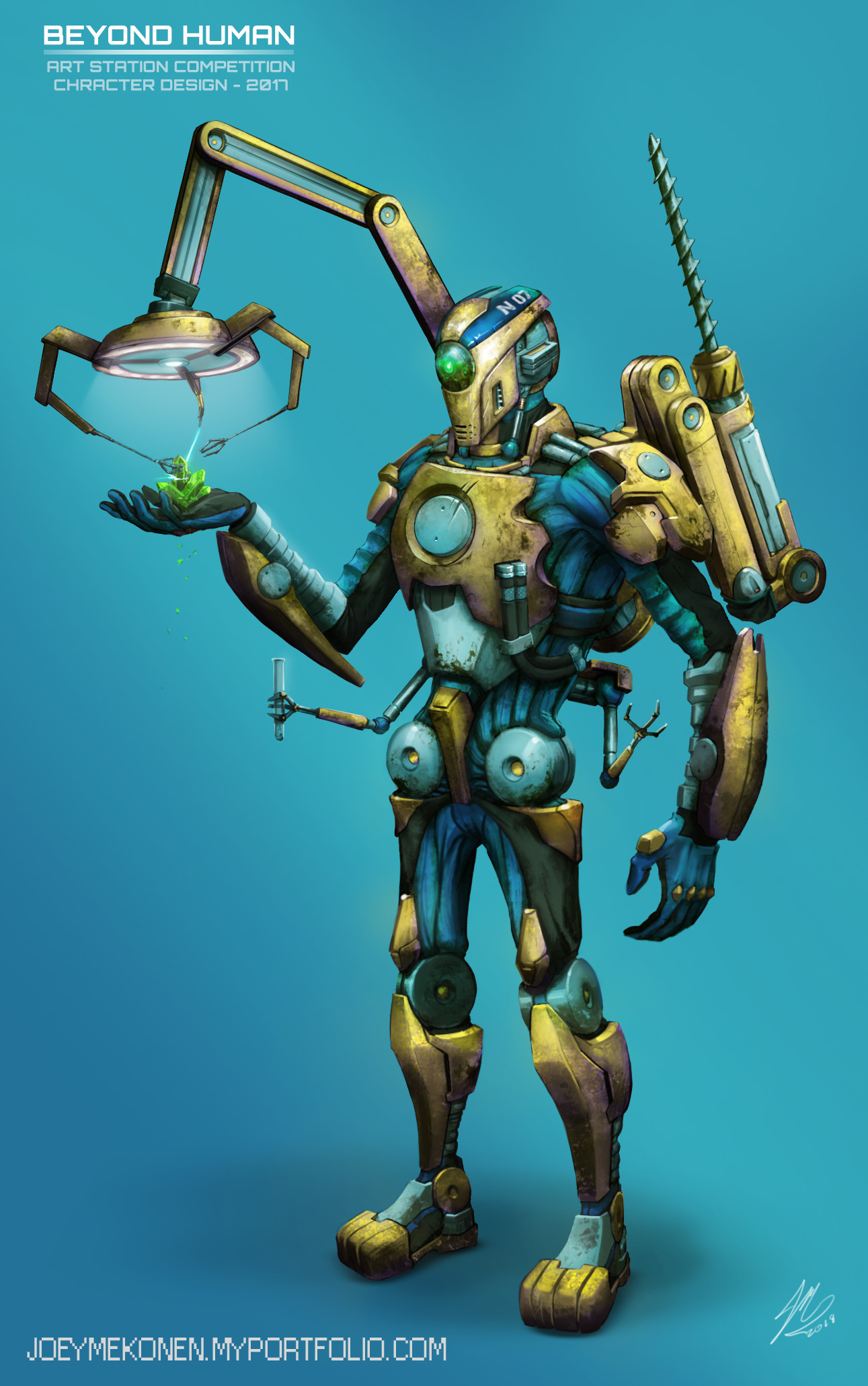The image depicts a meticulously detailed, computer-generated robot, possibly a superhero, set against a light blue background. Dominating the top left corner, white text reads "Beyond Human, Art Station Competition, Character Design 2017." In the bottom left, white text displays "joeymekonen.myportfolio.com," with a small, indistinct signature on the bottom right. The robot itself is clad in gold and blue armor, featuring notable elements such as a large green circular eye and small robotic arms emerging from its waist—one holding a knife-like tool. A bar extends from its back, terminating in a spotlight with three tiny feelers interacting with a green jewel in its hand, likely being shaped using lasers. Additionally, a drill and a utility pack are attached to its back, enriching the intricate design.